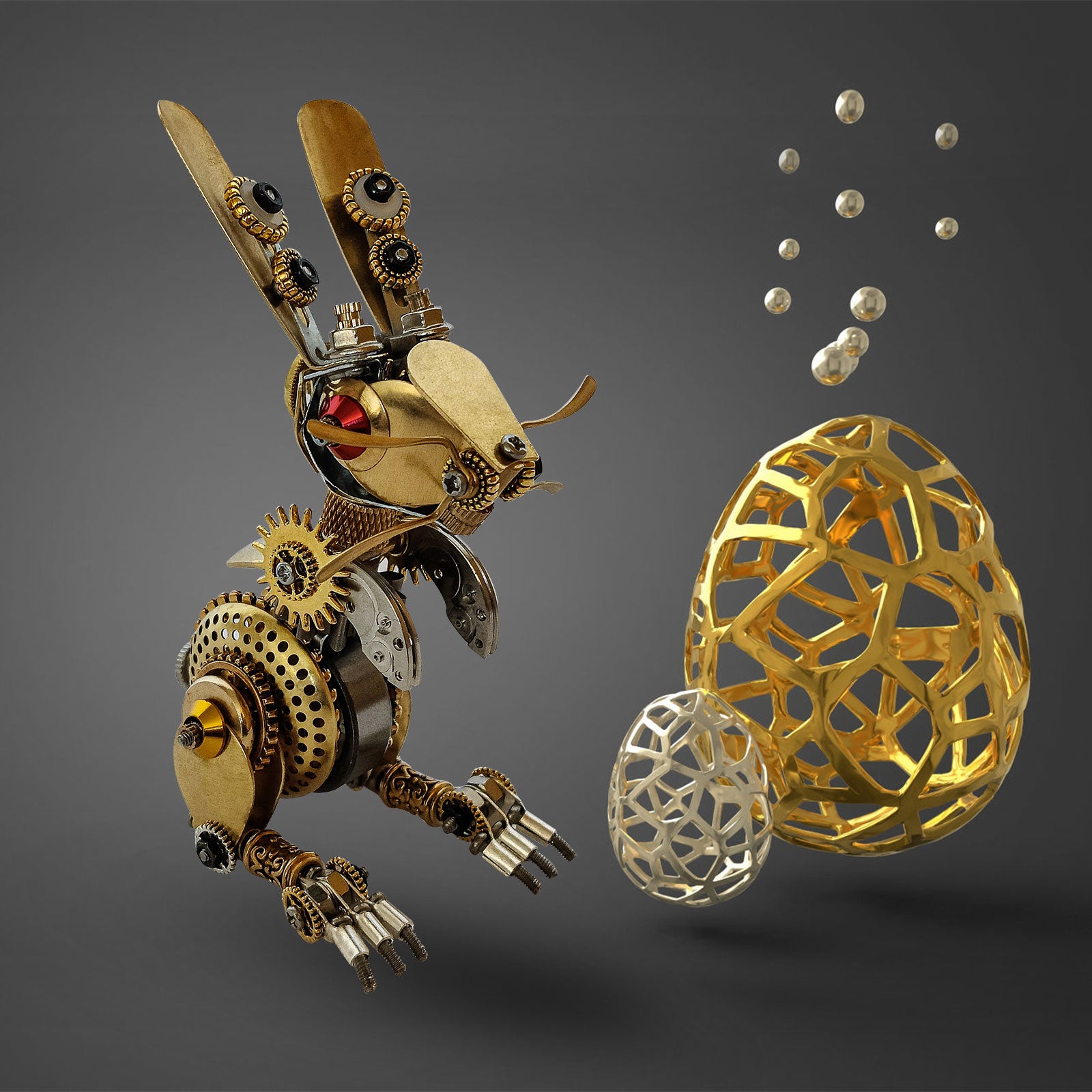The image showcases a mechanical, steampunk-inspired bunny rabbit adorned with intricate gears and cogs, primarily in shades of bronze, gold, and silver. The bunny features prominent golden ears with two circular knobs aligned in gold at the tips, as well as a striking red eye encircled by metallic elements. Further detailing includes small gold whiskers. Positioned on the right side of the image are two floating eggs—a larger golden egg comprised of a grid-like structure and a smaller, similarly constructed silver egg. Both eggs are designed with numerous holes that allow a glimpse of the plain, medium-dark gray background. Above these eggs, approximately ten shiny, small silver spheres are suspended in the air. The bunny appears broadside, with elements like fan blade-like ears and a doorknob handle protruding from its red eye, adding to its fantastical and whimsical mechanical design.